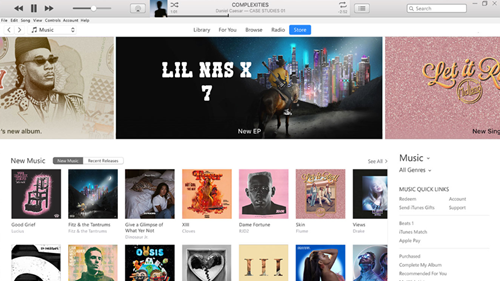A detailed caption for the image described would be:

The image displays an open iTunes window with a predominantly grey background. At the top, there's a typical music player interface featuring navigation icons: a black double arrow pointing left for 'previous,' a 'pause' icon with two vertical lines, and a double arrow pointing right for 'next.' The volume slider appears to be halfway filled. 

Black text highlights the complimenting sections, though the album name is illegible. The elapsed time of the song and the overall track length are indicated on the left and right sides, respectively, but the specifics are unclear. A white search bar is positioned on the right-hand side of the interface.

At the very top, a slightly lighter grey menu displays options: File, Edit, Song, View, Control, a menu that begins with 'A', and Help. Below this menu, on a white strip, navigation arrows point left and right next to a music note icon followed by the text "Music." The center of the interface highlights navigation tabs labeled "Library," "For You," "Browse," "Radio," and a blue "Store" button with white text.

In the center, the largest album artwork displayed belongs to Lil Nas X's "7 EP," indicated by the text "EP" at the bottom of the cover. Surrounding this, various other album covers for new music are shown, though the specific albums are not recognized.

On the right-hand side, a grey section contains listings under "Music," with filters for "All Genres" and "Quick Links," accompanied by smaller white and grey texts that are partially unreadable due to image sizing constraints.